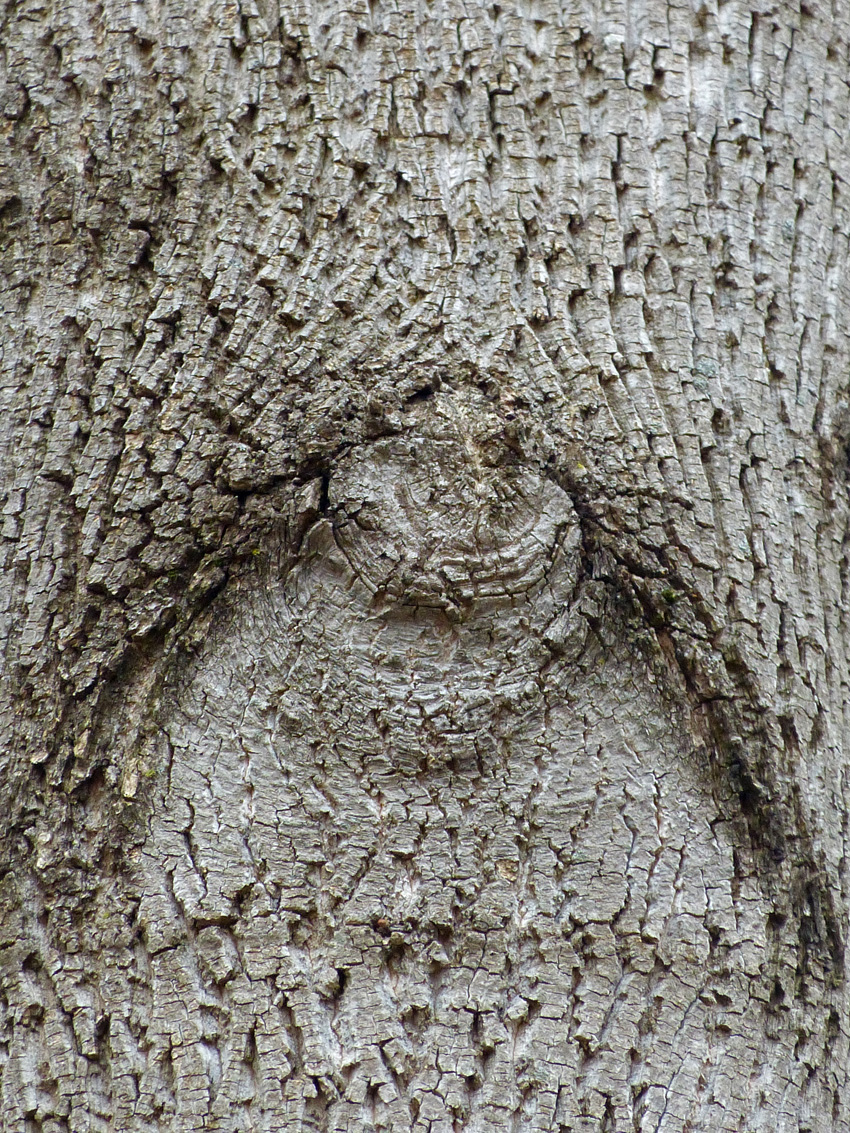This is a poster-sized, close-up image of a gray tree trunk, revealing its rough, deeply-indented bark. The bark's color varies from light gray to nearly white, with occasional hints of black, creating a complex, textured appearance. In the center of the image, a prominent knot is visible. From this knot, a semicircular depression fans out, with the flat side of the semicircle at the bottom. The depression and the knot together give the tree a distinct, tree-like appearance, almost resembling a V or arch shape. The bark appears rugged and jagged, filled with numerous small notches and indentations, giving it a highly detailed and tactile texture. The image is tightly cropped, focusing solely on the trunk and bark, excluding any branches or surrounding elements. This close-up view emphasizes the intricate natural patterns and textures of the tree's surface.